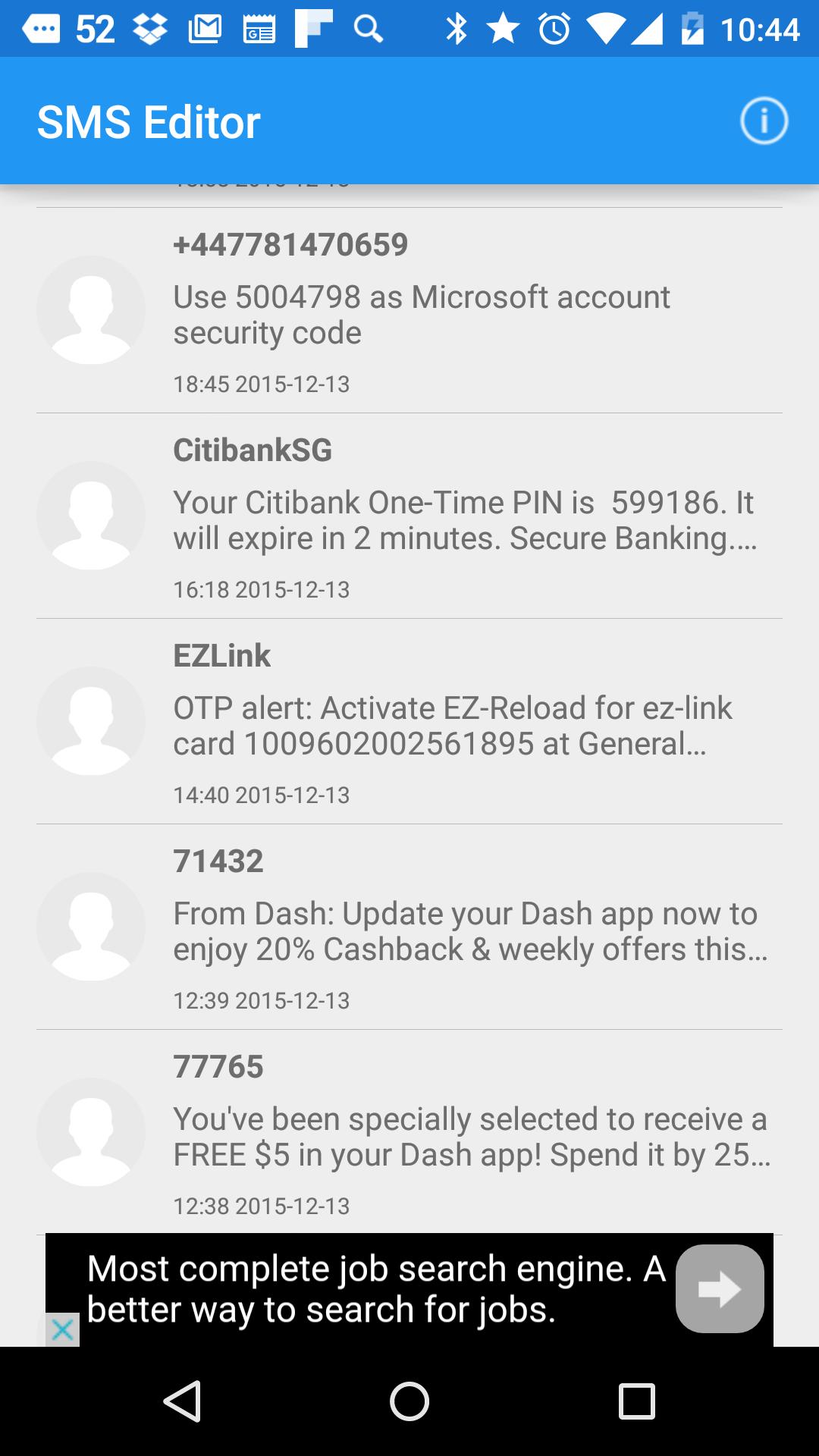The image is a screenshot of a cell phone display. At the top, there is a darker blue status bar featuring several icons: a left-pointing arrow, the number 52, an open box (likely Google Mail), the Google ID icon, an airplane resembling a B-52, a magnifying glass (search), Bluetooth, a star, an alarm clock, full cell signal, full service indicator, and a charging battery at 50%. The time shown is 10:44. Below this, there is a section with a light blue background and white text stating "SMS Editor." To the right, there is a circle with an "i" (information).

The main area of the screenshot has a gray background with various notifications and texts. One is from the phone number +44-77-81-47-06-59, stating "Use 547-98 as a Microsoft account security code." Another message from Citibank SG mentions, "Your one-time PIN is 599-186, it will expire in two minutes." EasyLink has sent a message from the number 74. There's also a text from 74-47-14-32 promoting "20% cash back on Dash App." Additionally, a message from 777-65 says, "You've been specially solicited for a free $5 on Dash App by spending $25." At the bottom, there is an advertisement with a black background and white text stating "Most complete job search engine, a better way."

The bottom navigation bar features icons in black: a triangle pointing to the left, a circle, and a square.